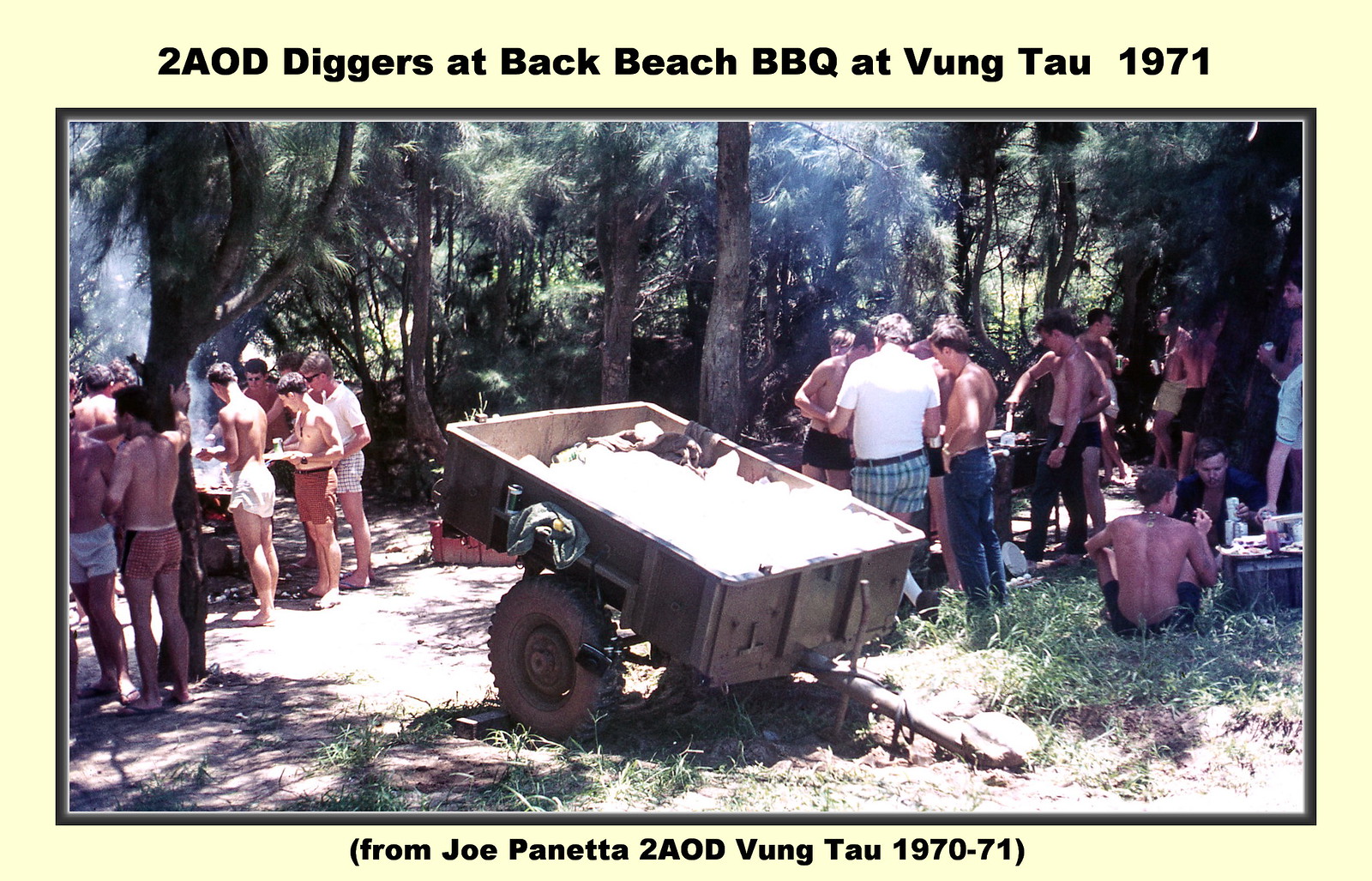This 1970s photograph, measuring approximately six inches wide by four inches tall, captures an outdoor scene at Vung Tau during the Back Beach BBQ in 1971. The image features a light cream-colored border with bold black text at the top reading "2AOD Diggers at Back Beach BBQ at Vung Tau 1971," and a footer with the text "From Joe Panetta to AOD Vung Tau 1970-71" in parentheses. The photograph itself is surrounded by a thin light gray border.

At the center of the photo is a single-axle, two-wheel trailer lying on its hitch, suggestive of a container typically pulled by a military vehicle. The setting is a mix of sandy and grassy areas, framed by tall trees typical of a jungle environment. Scattered throughout the scene are groups of white men, most of whom are shirtless and wearing swim trunks, indicative of a casual picnic or beach outing. Some of the men stand around barbecue setups, while others are seated at tables, enjoying their meals. The atmosphere is relaxed and communal, reflecting a day of leisure and camaraderie amid the lush, green backdrop of Vung Tau.